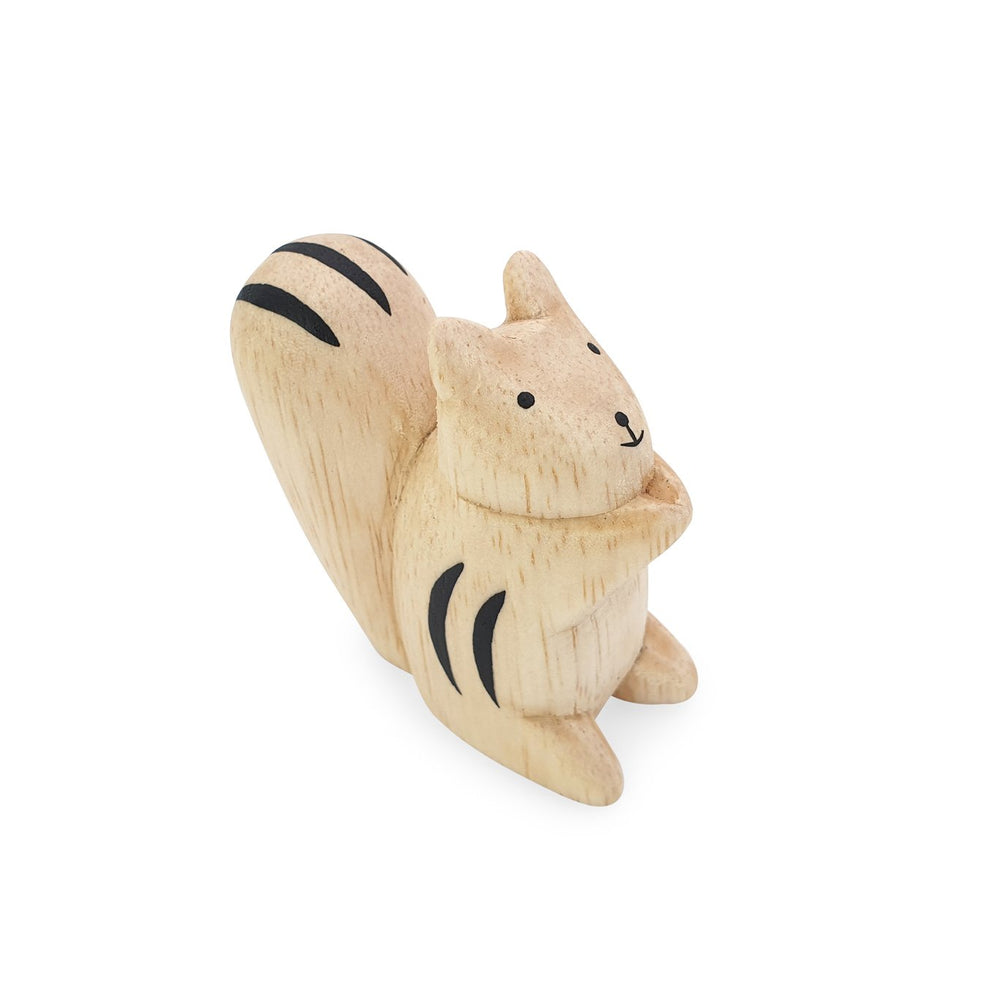The image features a charming, hand-carved wooden figure that appears to be a squirrel or perhaps a chipmunk, set against a plain white background. The small figure, crafted from very light tan wood with visible grain, has a simple yet endearing design, giving it the appearance of a child's toy. Its body is adorned with black painted details, including two eyes, a nose, a little smiling mouth, three stripes on its raised tail, and a couple of black stripes on either side of its body. The figure faces slightly to the right, with its tiny ears sticking up and its small paws positioned together in front of its face, resembling a praying posture. The figure's cute, chubby form and minimalistic coloration emphasize its handcrafted aesthetic, making it a delightful piece of art.